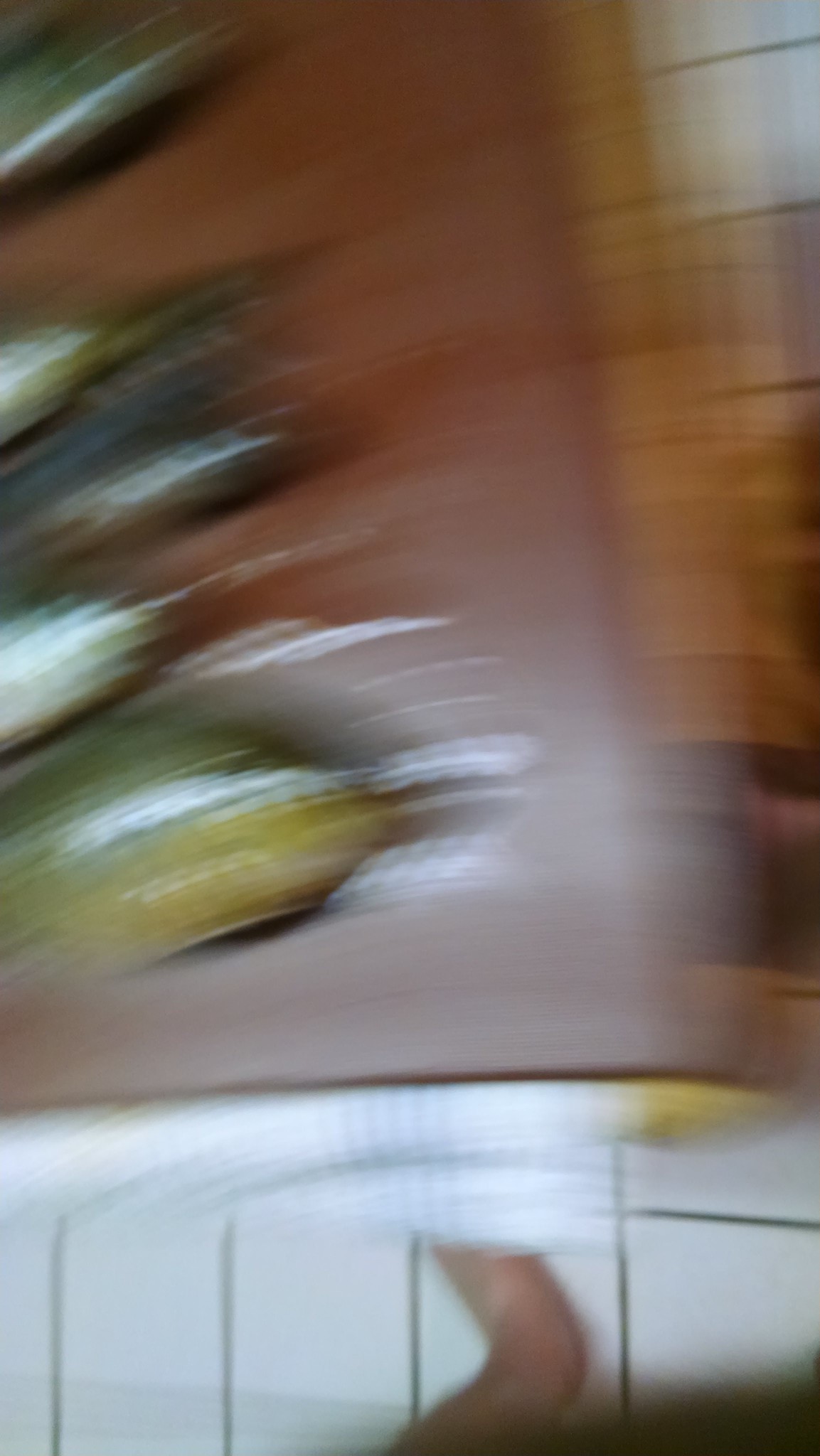This blurred image features a section of white rectangular floor tiles with black grout lines, partially occupied by an unidentifiable body part near the bottom edge. In front of these tiles, a white vertical line appears, accented with a touch of yellow on its right side. Moving upward from the yellow, the vertical gradient shifts to orange, then back to white, which might represent a continuation of the tiled flooring, though blurred. In the top right corner, the same white tiles with black grout lines can be seen again. To the left of the image is a red-bordered object, adorned with four circular items varying in color, including shades of yellow, white, green, and blue.